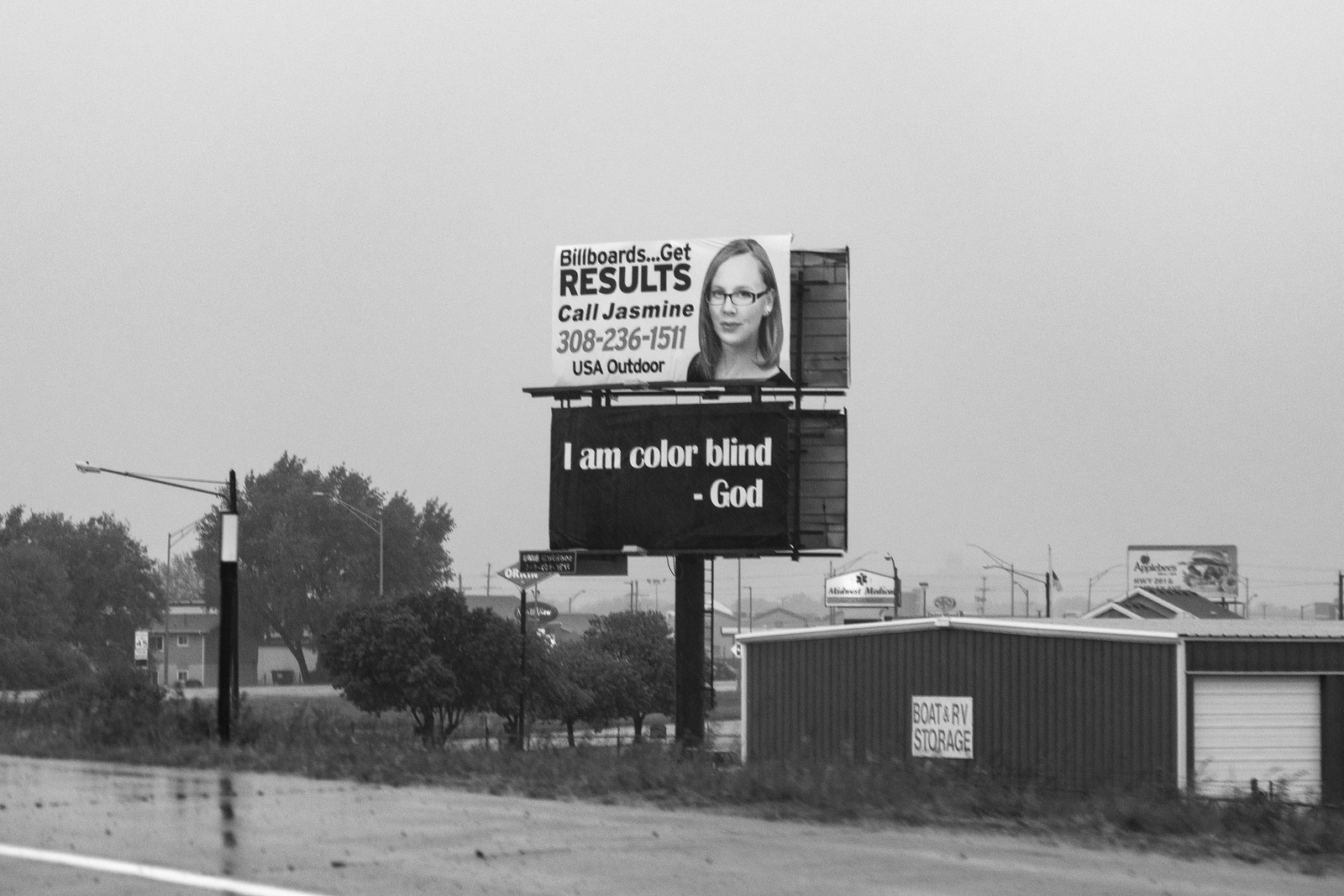This black-and-white photograph, taken in a rectangular landscape format, captures a roadside scene featuring two prominent billboards. The upper billboard advertises with the slogan, "Billboards, Get Results," followed by a call-to-action to contact Jasmine, inclusive of a phone number and a portrait of a woman. Just beneath it, a striking black-background billboard with white text displays the message, "I am colorblind," attributed to God. In the mid-ground, a large building prominently bears the signage, "Boat and RV Storage." The background reveals an array of trees interspersed with additional businesses and buildings, which trail off toward the right side of the image, encapsulating a blend of commercial and natural elements within the same frame.